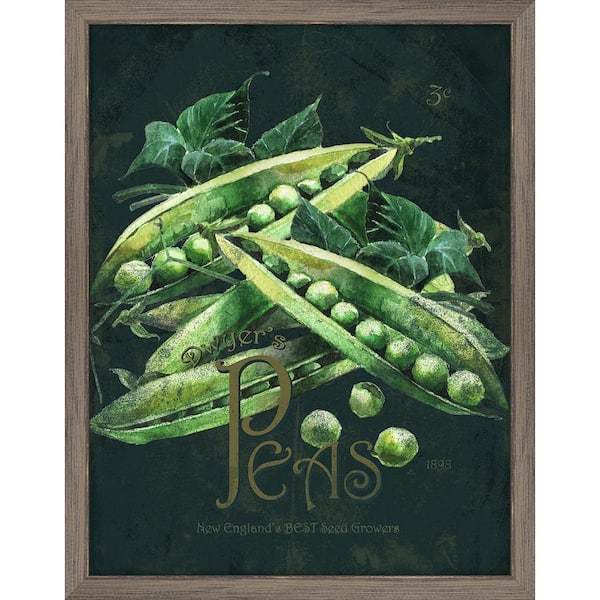This is a detailed illustration depicting "Dwyer's Peas, New England's Best Seed Growers" in bold text, prominently displayed above and below the main image. The painting, framed by a dark gray border, features a striking black background that contrasts with the lush greens of the pea plants. The pea pods, illustrated in a lighter green with a hint of yellow, reveal the vibrant peas inside, some spilling out in a lively manner. The leaves, a darker green, are intricately detailed with three distinct parts each, adding depth and texture. The composition shows several pods, some fully open and others partially closed, arranged in a natural, overlapping fashion, interspersed with vine leaves. The artwork beautifully captures the essence of fresh, enticing peas, evoking a sense of their delicious potential.